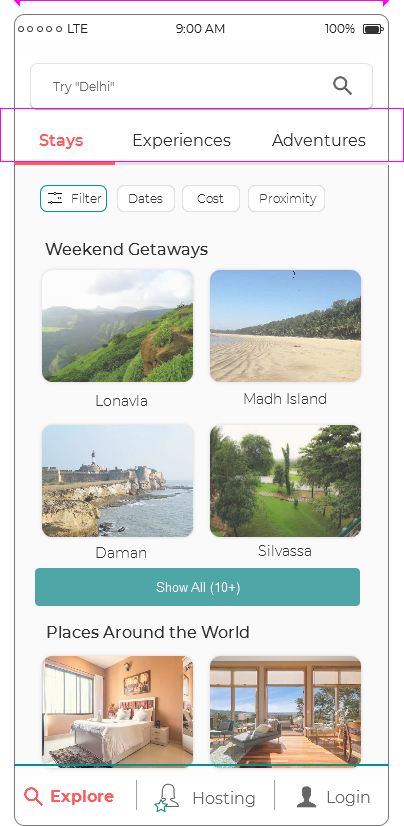This is a screenshot of a mobile app interface. At the very top, there is a purple line, alongside status icons indicating a fully charged battery at 100%, the time at 9 a.m., LTE connectivity, and four signal bars. Below this, there is a large search bar with a purple outline. Surrounding the search bar, you can see several navigation options in red text: "Stays," "Experiences," "Adventure," "Filter," "Dates," "Proximity," and "Weekend Getaways."

Below these options, there are four thumbnail images showcasing various weekend getaway destinations. Each image has descriptive text:
- The first image shows the iconic "Moai Island Head," featuring sand, mountains, and a blue sky.
- The second picture depicts a landscape with "Long Via," highlighting rays of mountains and lush greenery.
- The third image is labeled "Mine" and shows a coastal lighthouse.
- The fourth photo, marked "Syl Vasa," presents a picturesque landscape.

Beneath these images, there's a green bar that reads "Show all ten."

Further down, a section titled "Places Around the World" catches the eye with options to "Explore" (written in red), "Hosting" (marked with a blue star next to a silhouette person icon), and "Login" (featuring a person silhouette). Below this section, two additional images are shown: one of a bedroom and the other offering a scenic window view.